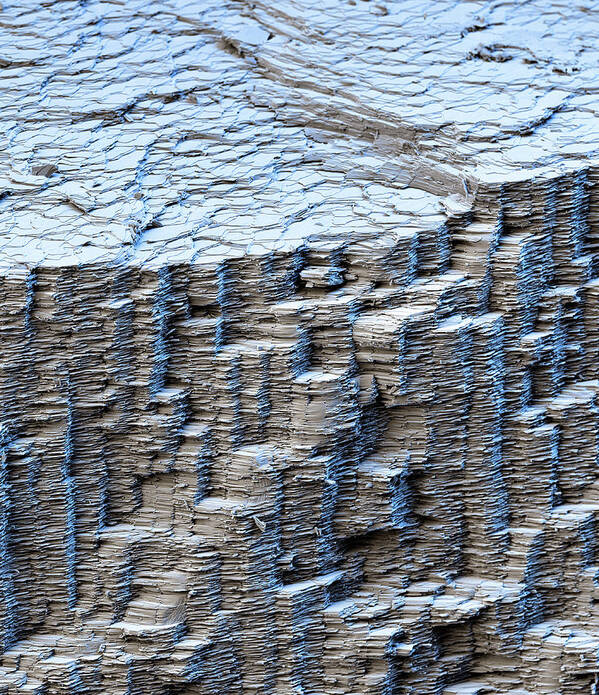This image shows an up-close view of a textured, layered rock formation. The rocks appear to be stacked in thin, jagged slabs reminiscent of cardboard or paper, with their edges sharply uneven. The rock formation's side is a dark gray or slightly darker brown, presenting a staggered, almost staircase-like appearance. On top, the formation is lighter and features raised, circular patterns akin to alligator skin, which reflect light and give it a metallic silver or shiny look. The detailed layers and intricate textures emphasize the unique geological structure of the rock.